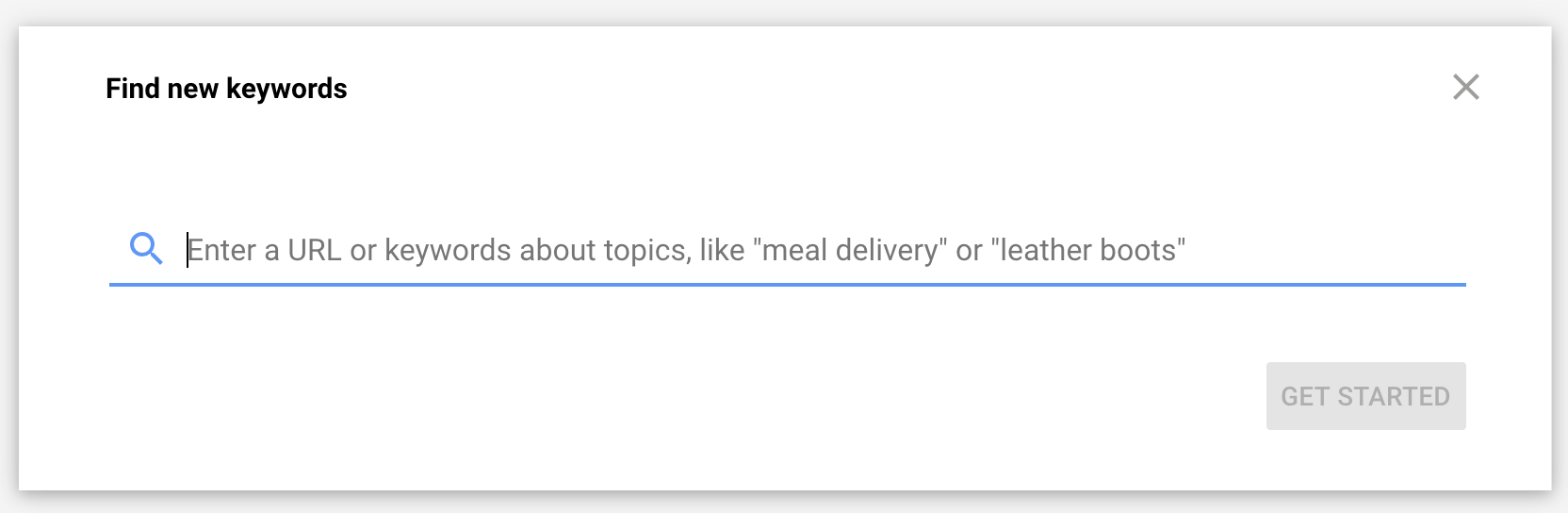The image is a small, cropped screenshot showcasing a search interface. At the top, in black font, there's the text "Find New Keywords." Directly beneath this title is a blue magnifying glass icon, accompanied by a blue underline indicating where you can enter a search prompt. Above the blue underline, in gray text, are placeholder instructions that read: "Enter a URL or keywords about topics like 'meal delivery' or 'leather boots'." On the bottom right corner of the interface, there's a gray button labeled "Get Started." Additionally, in the upper right corner of the image, there's a gray 'X' icon, which can be clicked to close the prompt. This interface appears to be a search feature, designed to find information based on a URL or specific keywords, although it is unclear whether it is for a document search or a broader search engine.